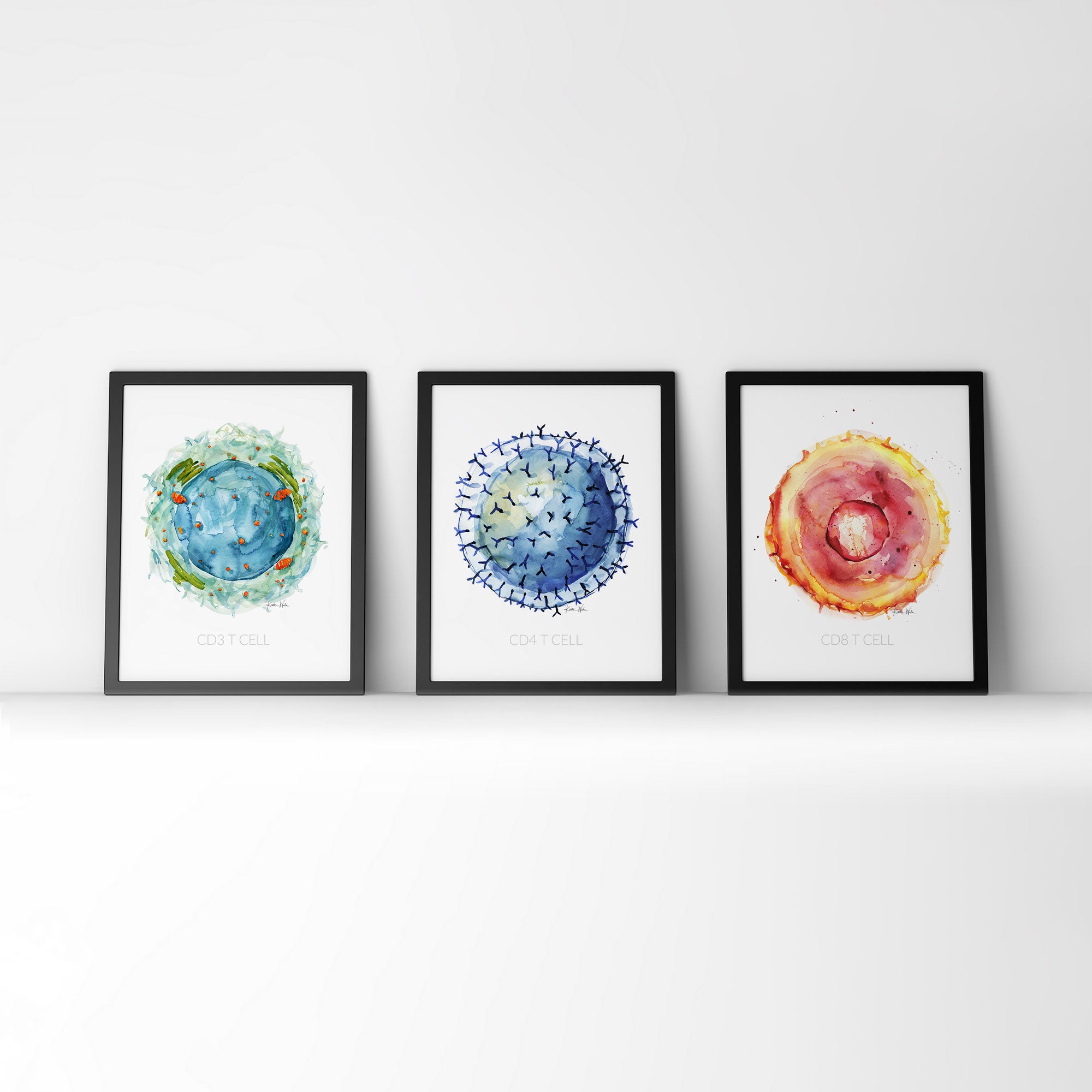The image features three scientifically illustrated portraits, each in identical black frames, propped against a white wall on a white surface. Each portrait is vertically oriented, taller than it is wide. The first portrait on the left, labeled “CD3 T cell,” depicts a blue circular form, resembling a planet with orange and green elements orbiting it and a greenish halo. The second portrait in the center, labeled “CD4 T cell,” shows a blue circle with darker blue, almost black, and medium blue spikes or specks protruding from it, ringed by a more defined blue halo. The third portrait on the right, labeled “CD8 T cell,” presents a vibrant red circle with a mixed red and white nucleus and a yellow-orange periphery, dotted with small black specks. All three portraits appear to be created using watercolor technique.